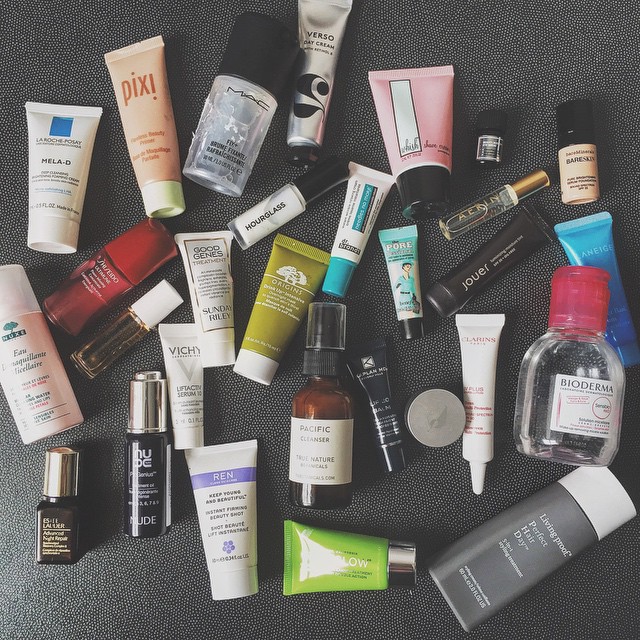Caption: A meticulously arranged assortment of travel-sized beauty products is displayed on a lightly speckled, textured surface. The surface features a subtle pattern of small black and gray dots, discernible only upon close inspection. The collection includes a variety of containers, ranging in size and shape, from round to square, with none exceeding two ounces in volume. The bottles and jars are vividly multicolored, each sporting unique labels and designs, adding a burst of visual interest. The mix includes both plastic and glass containers, representing an array of different manufacturers, showcasing a diverse selection of beauty essentials ideal for on-the-go use.